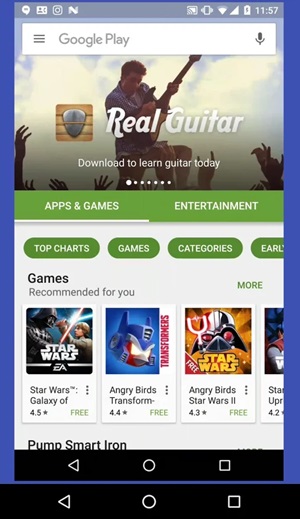The image presents a vivid and dynamic layout of a mobile screen interface, captured in detail from the top to the bottom:

In the top left corner, the blue background contrasts with a series of icons including a bubble, a square, the Instagram logo, a large square with wave-like patterns, a vibrating square, the Wi-Fi signal indicator, a large signal bar, and a battery icon showing a charge status of 11:57. Below these icons is a wide Google Play search bar that includes a microphone icon. The text reads "Light the Light".

Just below, the app "Real Guitar" is prominently displayed. The app's icon features a striking image of a black and blue dragon alongside a large guitarist playing a guitar in front of a brown wooden background. A guitar pick is visible in the foreground, while in the background there are numerous raised hands, evoking the energy of a live concert. The accompanying text encourages users with "Download to learn guitar today". 

The interface includes a series of navigation circles—numbered 1 through 7—with a green bar highlighting the active section. The white text on the green bar identifies various categories such as "Apps and Games" and "Entertainment", with an oval button labeled "Top Charts". Other categories listed include "Games" and "Recommended for You".

Featured prominently within these categories are several applications, including the "Star Wars" themed games. Iconic characters like Vader and Luke are depicted, promoting games such as "Star Wars Galaxian", "Angry Birds Transformers", "Angry Birds Star Wars 2". The screenshot further lists sequels "Star Wars 4, 5, 6", mentions the phrase "This pumps my iron", and lastly it includes a subtle gray text at the bottom.

The visual complexity and diversity of elements cohesively convey an interactive and engaging mobile screen experience.